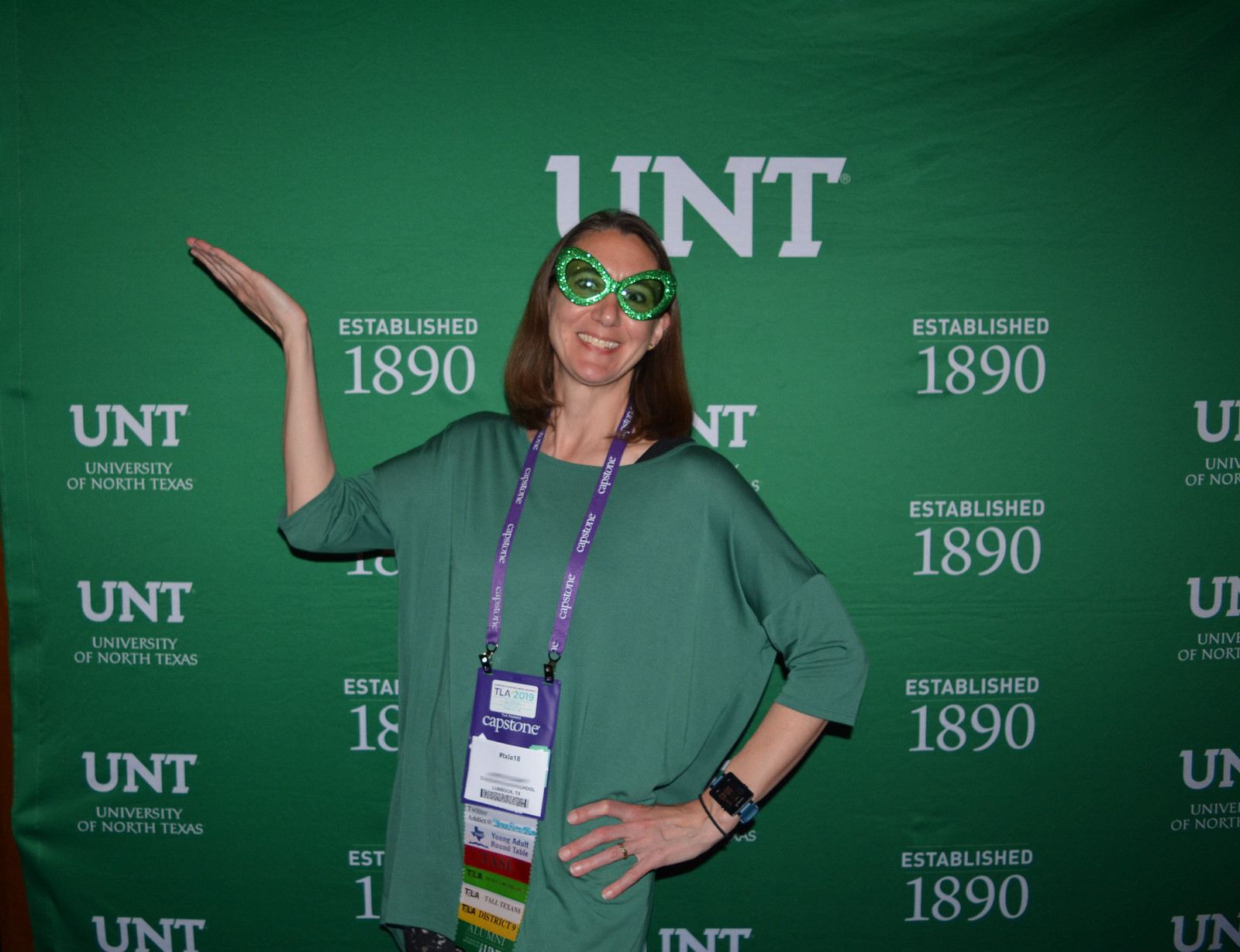This detailed photograph captures a woman standing in front of a vibrant green backdrop adorned with the University of North Texas (UNT) logo and the phrase "Established 1890" repeatedly in white text. The woman is dressed in a matching green shirt and is sporting oversized, sparkly green novelty sunglasses. She raises her right hand with her palm facing outward. Around her neck, she wears a ribbon with a series of badges; the most prominent is a large purple one reading "Capstone," followed by several smaller badges in white, red, green, yellow, and other colors, displaying variations of the acronym "TASE." The setting appears to be a UNT event, possibly for alumni, with the uniform green backdrop and repeated UNT branding suggesting an official photography area. The woman also wears what appears to be a smartwatch on her wrist, adding a modern touch to her ensemble.